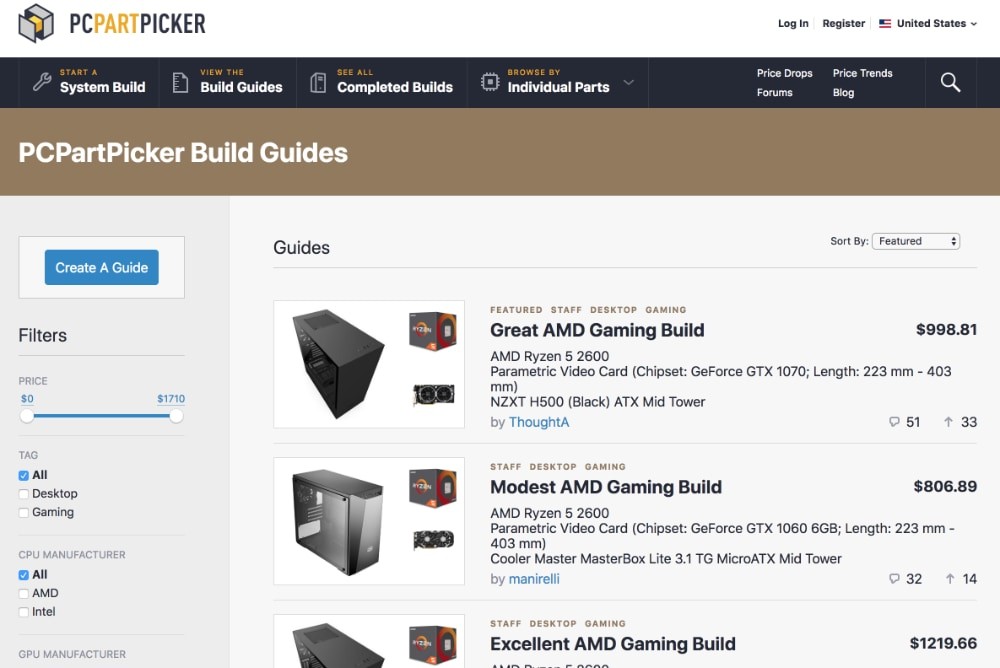A screenshot of the PC Part Picker website is captured in this image. In the upper left corner, the PC Part Picker logo, a square resembling a single drawer of a cabinet or possibly a bolt, is displayed. The top menu bar, a very dark blue, features several navigation options: "Start a System Build," "View the Build Guidelines," "See All Completed Builds," and "Browse Individual Parts," the latter of which includes a drop-down menu.

In the upper right corner, against a white background, there are three black-lettered links: "Log In," "Register," and an option to pick the user's location. Here, the location is set to the United States, indicated by a small adjacent flag.

The secondary menu bar below the main one is a dark brown rectangle with white text, reading "PC Part Picker Build Guides." Directly beneath this, the body of the website displays a selection of PC parts. The highlighted build on top is the "Great AMD Gaming Build," priced at $998.81.